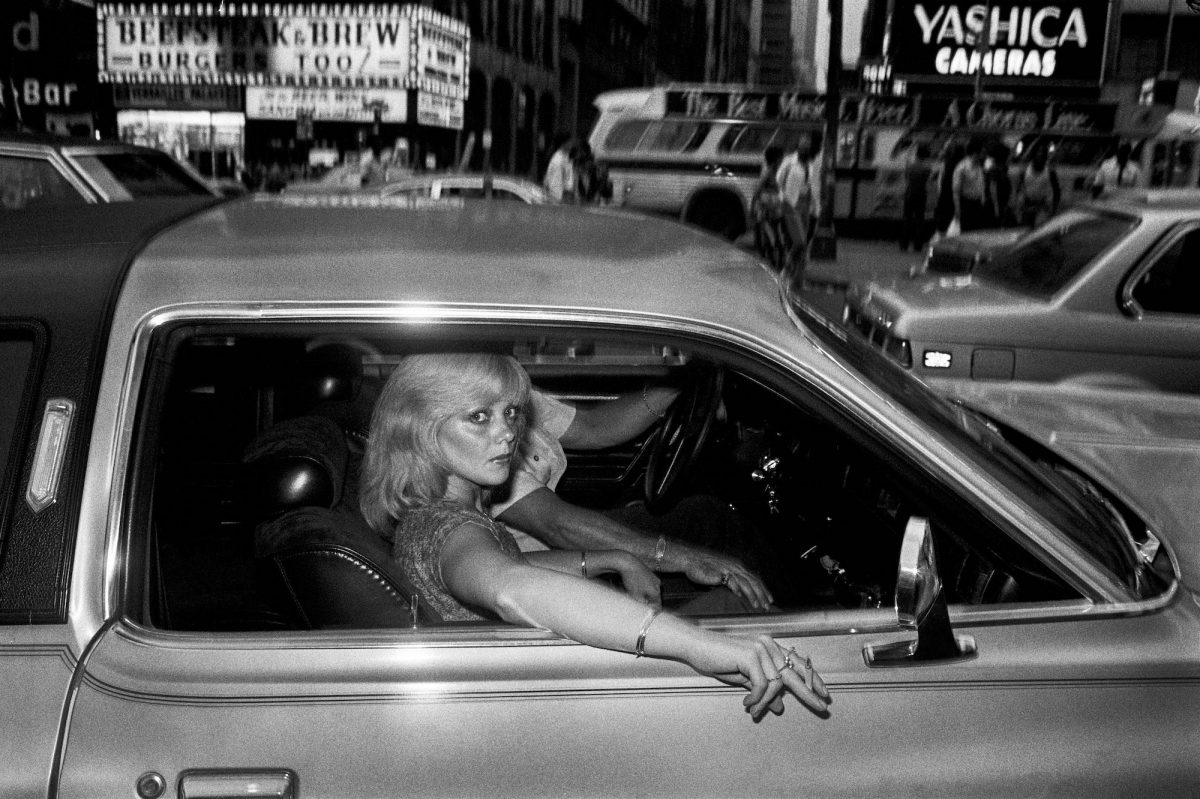In this detailed black-and-white photograph, an outdoor nighttime scene on a bustling city street is depicted. The central focus is a seemingly silver car with a blonde, attractive Caucasian woman sitting inside, gazing out of the window. She has big eyes, wears a short-sleeved shirt, and adorns her right wrist with a bracelet. She holds a cigarette between her fingers, with several rings visible on her right hand. Next to her in the driver’s seat is a man, though his features are less distinct. The background reveals a blurred but clearly busy street, with numerous cars, people, and illuminated signage. Notable signs include "Beefsteak and Brew, Burgers Too" and "Yashica Cameras," contributing to the lively urban atmosphere. The image captures a classic, older time, encapsulated solely in shades of black and gray.